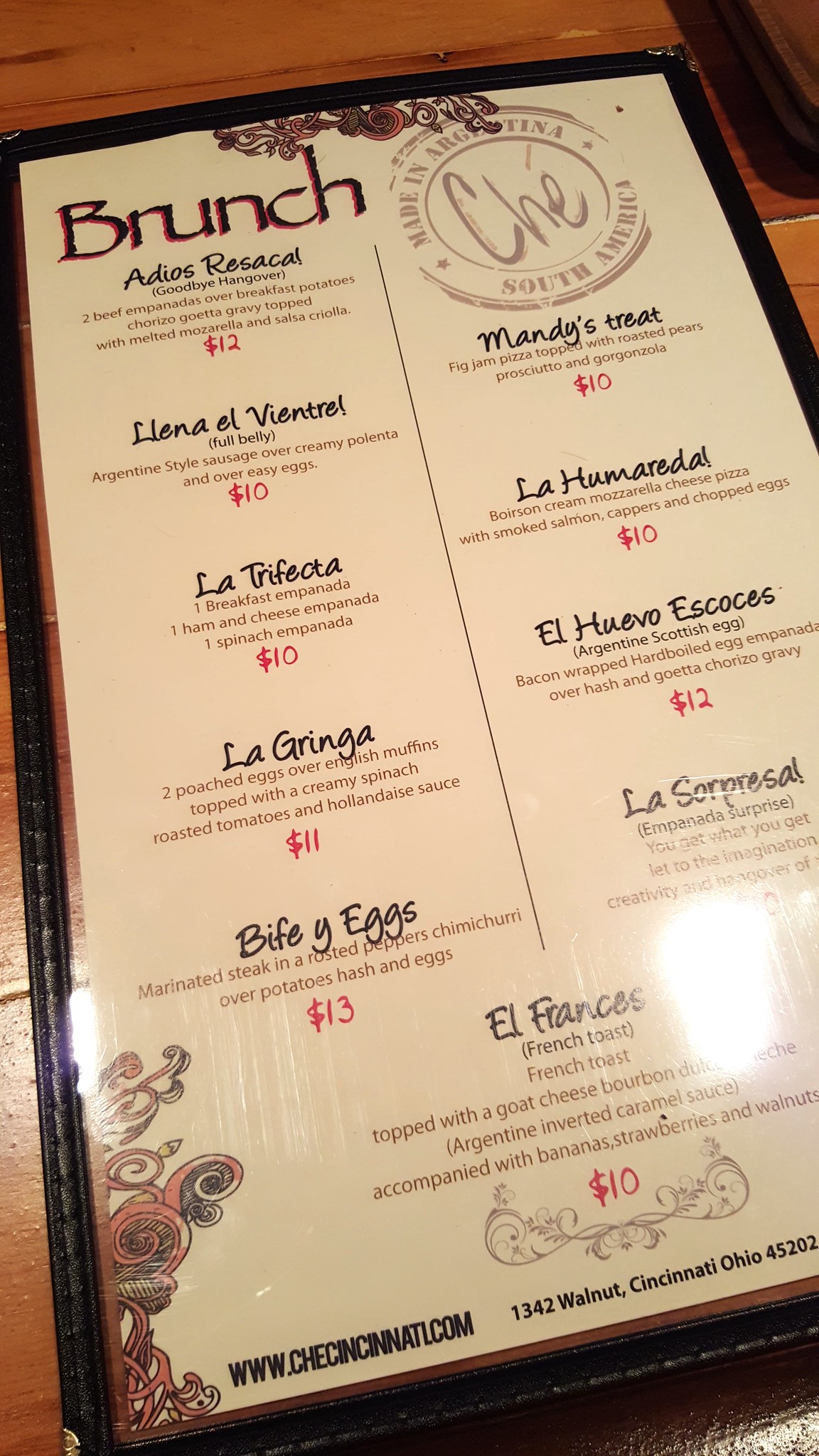A detailed photograph of a brunch menu placed on a rectangular plastic holder is seen resting on a light wooden table. The menu itself, bordered in black plastic, boasts a cream-colored background. In the upper right-hand corner, it prominently displays the name "Che" with the tagline "South America, made in Argentina." The word "Brunch" appears in dark reddish-brown lettering at the top left corner of the menu, under which various menu items are listed in Spanish. Featured dishes include "Adios Rosacao," "La Trifecta," "La Grinja," "El Huevo Escoces," among others, with a total of ten items listed. Notably, "El Frances," which translates to French toast, is mentioned at the bottom of the menu. Each dish is accompanied by a brief description with prices ranging from $10 to $13.